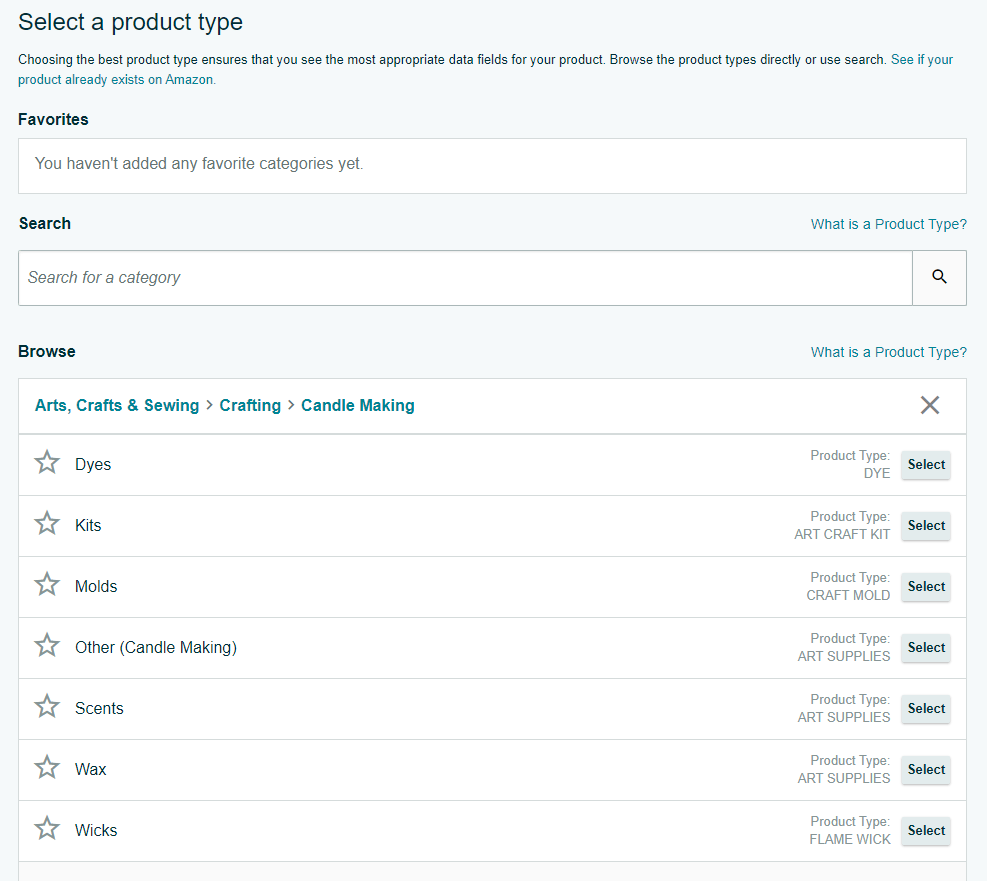The image showcases a user interface section for selecting a product type on a retail platform, likely Amazon. At the top, there's a prompt that reads, "Select Product Type," instructing users to choose the most appropriate category to ensure relevant data fields are displayed.

The interface allows users to browse product types directly or search for a specific product. If a product already exists on Amazon, it can be added to favorites. However, the "Favorites" section is empty, indicated by the message, "You haven't added any favorite categories yet."

Below the search bar, there is a browsing section titled "Arts, Crafts, and Sewing," with subcategories including "Crafting" and "Candle Making." The "Candle Making" section expands to list several items, each preceded by a star icon with a gray outline and white fill. The items listed are:

- Dyes
- Kits
- Molds
- Other Candle Making
- Scents
- Wax
- Wicks

Each item has an associated "Select" button for easy selection. 

On the right side, there is a series of drop-down options labeled "Select Product Type" with blue text asking, "What is a product type?" Multiple instances of these questions are displayed, suggesting the importance of selecting the correct category. The options include:

- Product Type: Die
- Product Type: Art Craft Kit
- Product Type: Craft Mold
- Product Type: Art Supplies
- Product Type: Flame Wick

Each option also features a "Select" button for choosing the specific product type relevant to the user's items. This detailed interface helps users categorize their products accurately, facilitating better organization and searchability on the platform.